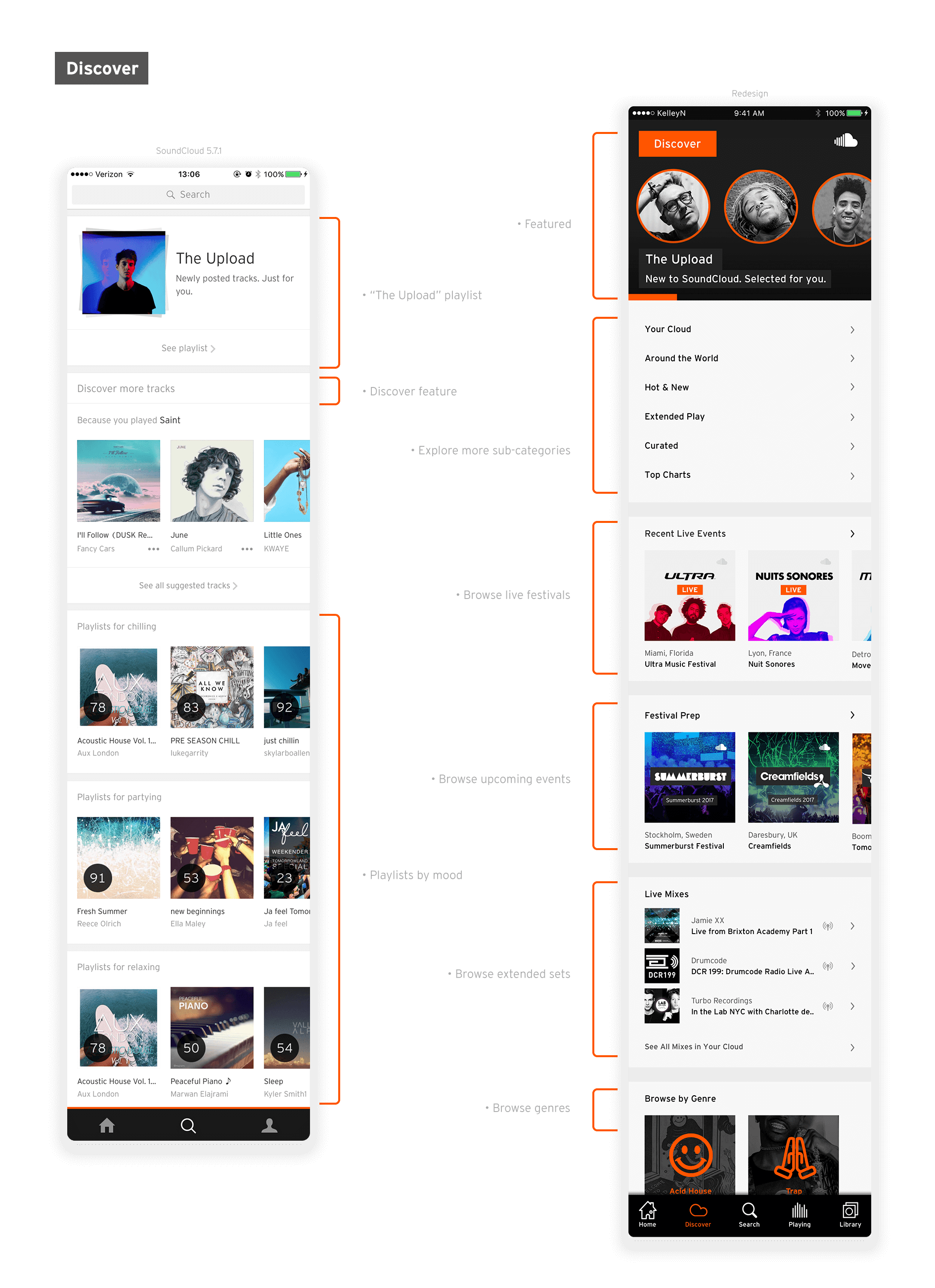**Detailed Caption:**

The image displays a comparative screenshot of two different mobile web interfaces, connected visually by thin red lines highlighting corresponding sections. In the center of the image, there are labels with white text on a black background, providing explanations for various segments of the interfaces.

On the left side, the first screenshot showcases a mobile webpage with a title at the top indicating "Upload." Beneath this, there is a picture featuring a man's head and shoulders, followed by a section labeled "Browse more tracks," which contains several album covers. The subsequent labels identify different features, starting with "Upload Playlist" at the top. As we move down, the labels show sections like "Discover Feature" and "Playlist by Mood."

The right side of the image presents another mobile webpage with circles at the top containing black and white headshots of individuals, alongside a discover button. The first label reads "Featured," followed by sections such as "New to SoundCloud" and "Selected for You." Below, a list of text appears with a label indicating "Explore More Subcategories." Further down, sections include "Recent Live Events" with a label "Browse Live Festivals," "Festival Prep" with colorful squares (blue and green) labeled "Browse Upcoming Events," "Live Mixes" labeled "Browse Extended Sets," and at the very bottom, a section labeled "Browse by Genre" indicating various musical genres.

The red lines between the sections allow for easy visual comparison of similar features across both webpages, making the structure and navigation paths clear.